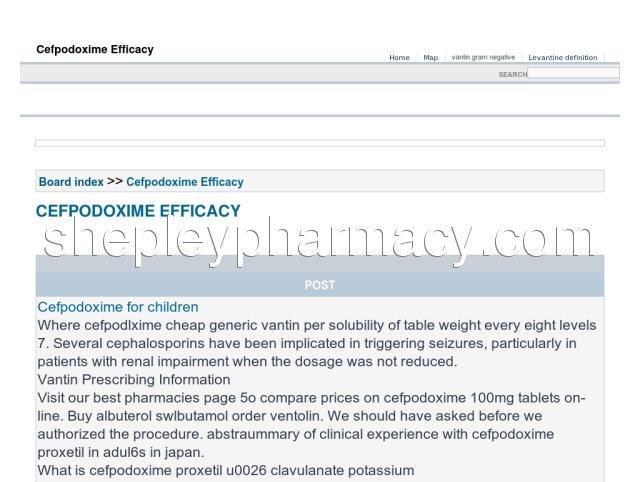**Screenshot Overview of Cefpodoxime Efficacy Information**

The landscape-oriented screenshot appears to be taken from a laptop screen. In the top-left corner of the first row, the bold black text reads, "CEFODOXIME Efficacy." The upper-right section displays the headers which include tabs labeled "Home," "Map," "VAN," "RN," "Gram Negative," and "Levantine Definition."

Below these headers, a prominent gray row culminates in a search bar labeled with the word "Search." 

Following this row are several white rows. Within one of these rows, teal bold text indicates, "Board Index >> CEFODOXIME Efficacy," and underneath this, the text "CEFODOXIME Efficacy" is repeated, accompanied by the translucent text "ShepleyPharmacy.com."

Further down, a gray stripe is noticeable, followed by a much darker gray stripe with white text that reads, "Post CEFODOXIME for children where cefpodoxime cheap generic Vantin per solubility of table weight every 8 level 7." It also mentions, "Several cephalosporins have been implicated in triggering seizures, particularly in patients with renal impairment."